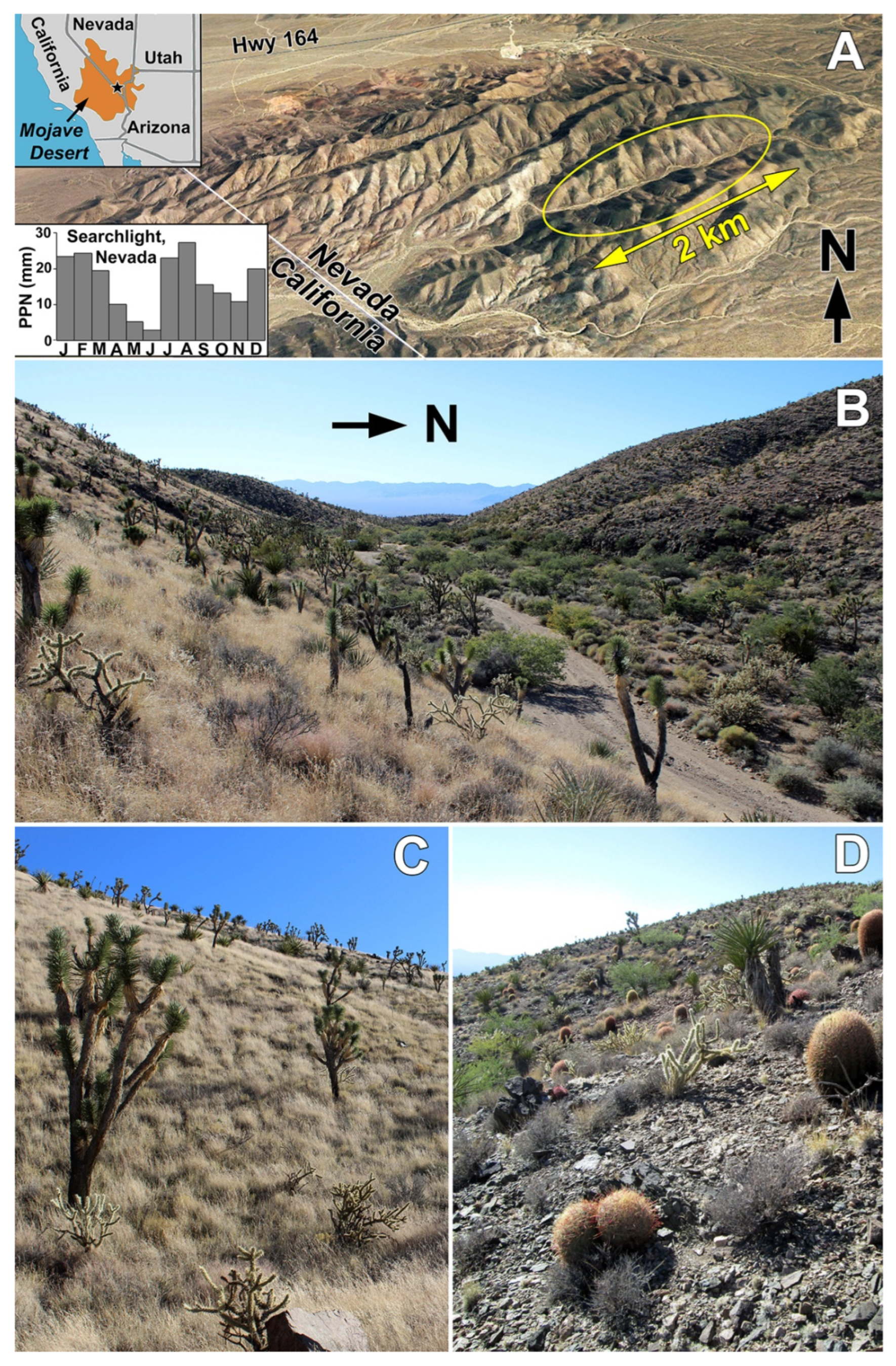This set of four images, marked A, B, C, and D, offers various perspectives of the Mojave Desert. Arranged in a vertical format, the top image (A) spreads horizontally like a postcard, illustrating the desert landscape at the California-Nevada border, complemented by an inset map of the Mojave Desert and a graph likely depicting rainfall across the year. The second image (B) presents a mountain range with an indication of how two kilometers appears in the area, featuring low desert scrub under a clear blue sky. The lower half of the set is split into two vertical sections: the third image (C) captures a valley intersected by a dirt road with mountains in the distance and a north direction marker pointing to the right, while the fourth image (D) shows a hillside adorned with barrel cacti. All four sections are enhanced with white letters in the upper right corners, and several images include indicators of cardinal directions, emphasizing the geographical context and variability within the desert landscape across California, Nevada, Arizona, and a portion of Utah.